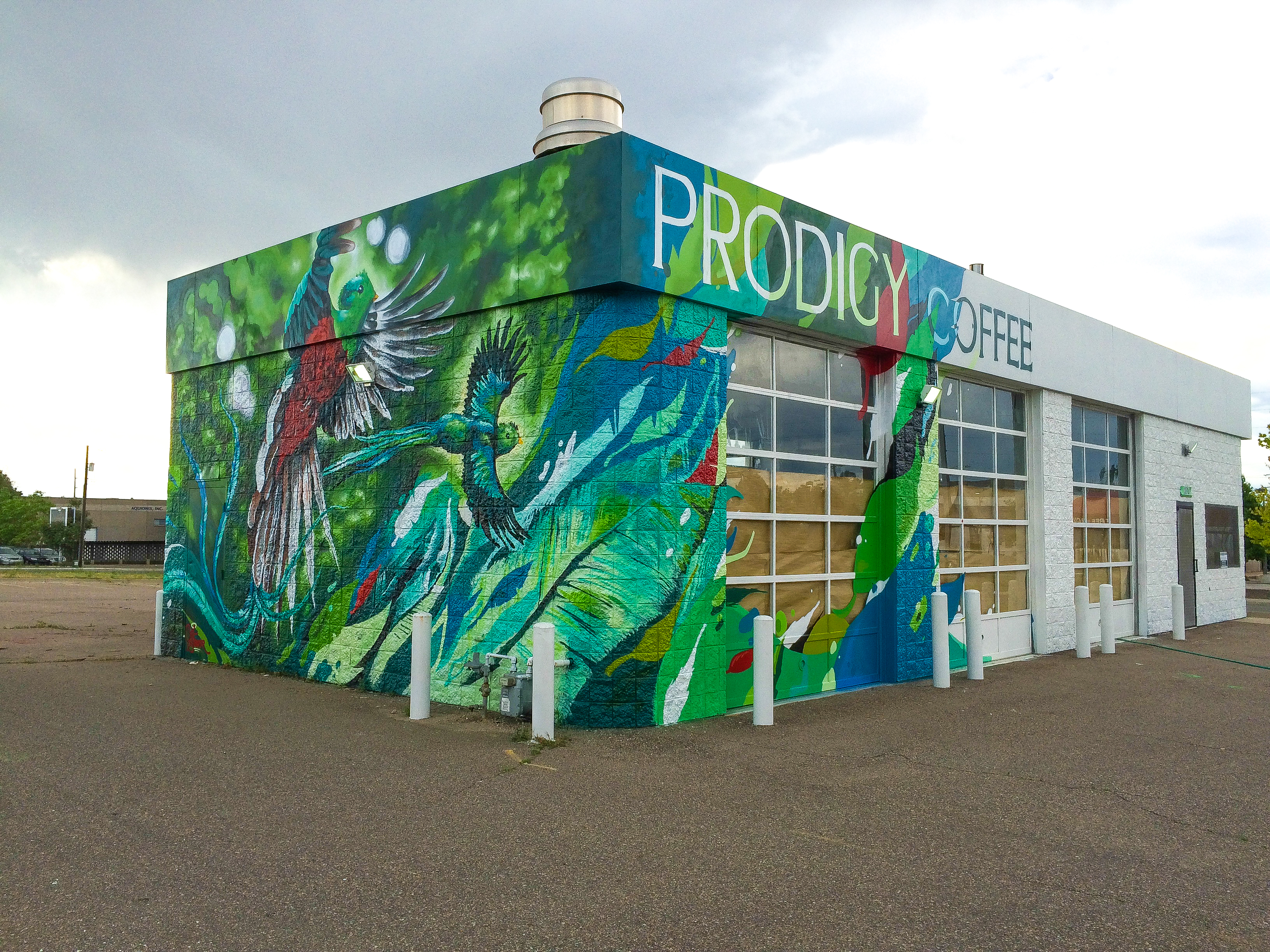This is a color photograph of a building that appears to be a repurposed gas station or oil change facility, now transformed into a coffee shop named "Prodigy Coffee." The building’s exterior is predominantly white, with impressive artistic features. Prominently on the left wall, there is a mural of two vividly colored birds against a forest green background. The bird on the left sports a green head, red body, and white feathers, while the bird on the right is green and black in mid-flight. The front façade of the building has three large garage doorways with glass windows and a smaller doorway to the right. The upper right section of the building features the word "Prodigy" in white text, with the word "Coffee" in blue and green text stretching over the garage doors. The building is surrounded by an asphalt parking lot. The sky above is partly cloudy with shades of white and gray, adding contrast to the vivid hues of the mural. This photograph captures the vibrant transformation and artistic flair of the establishment, highlighting the stunning mural and the structure's new purpose.